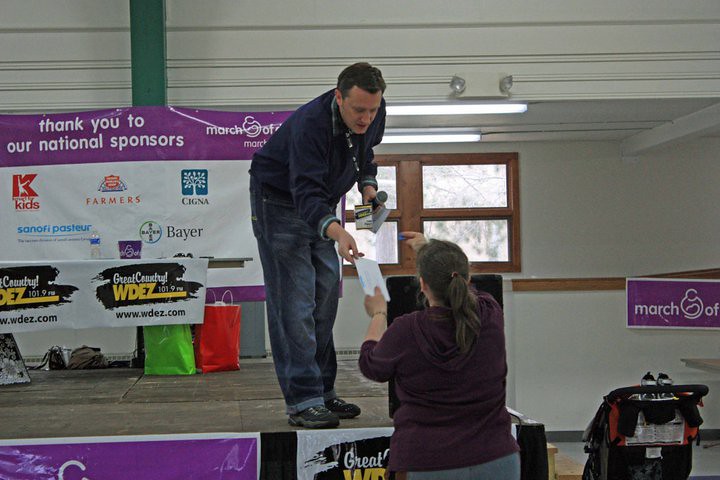In the image, a man in a blue sweater, blue jeans, and black shoes stands on a stage, holding a microphone in his left hand. He appears to be in his 30s or 40s and is wearing a badge. The man is handing a small piece of paper, possibly a letter, to a woman standing below the stage. The woman, facing away from the camera, is only partially visible; she is wearing a purple sweatshirt and has short hair. 

Behind the man, a large banner reads "Thank You to Our National Sponsors," displaying numerous company logos such as Farmer, Senha, Sanofi, Pasteur, and Bayer. Below this main banner, there is a table draped with another banner that reads "Great Country, WDEZ 100.9 FM," indicating that the event is likely associated with a radio station. To the left of the stage, there is a window showing a snow-covered landscape outside. Additionally, on the right side of the image, a small poster affixed to the wall displays the word "March." The scene is illuminated by white fluorescent lights, contributing to the indoor setting of what appears to be a formal gathering or radio event.